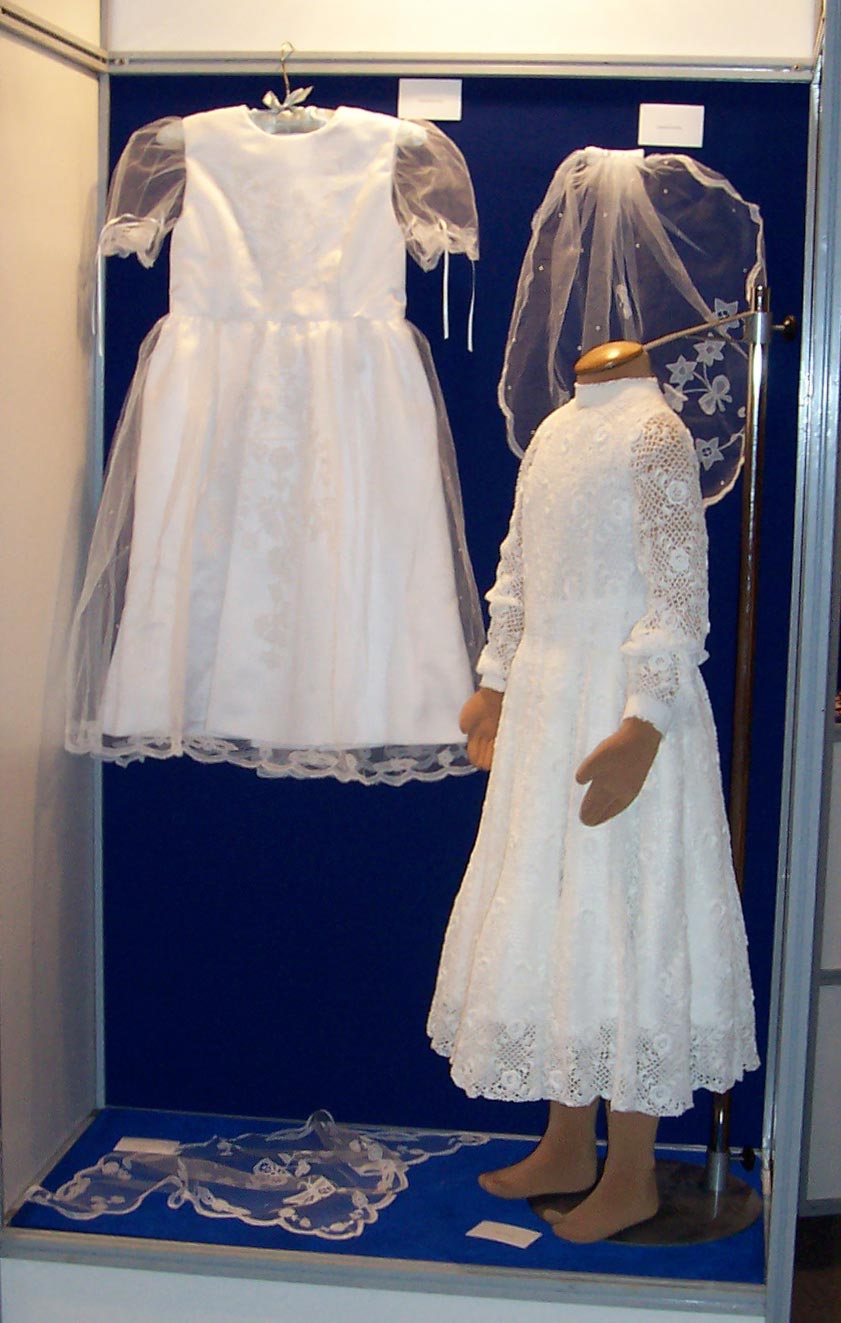This photograph captures a museum display featuring two meticulously crafted children's wedding dresses. Enclosed in a clear glass case with a royal blue background and flooring, the display showcases an ethereal ambiance. Hanging prominently at the top is a delicate white dress adorned with intricate sheer lace on its short sleeves and skirt, creating a whimsical and airy effect. To the right, a headless, small brown mannequin stands, turned slightly to the side, dressed in a similar but more elaborate long-sleeved white dress. This dress features rich lace detailing throughout, with the fabric extending to the sleeves and a solid white design embellishing the entire garment. Both dresses exude a timeless elegance, making it clear that they are designed for young girls, possibly for a wedding or ceremonial occasion. The silver walls frame the display, enhancing the sophisticated and historic atmosphere of the exhibit.